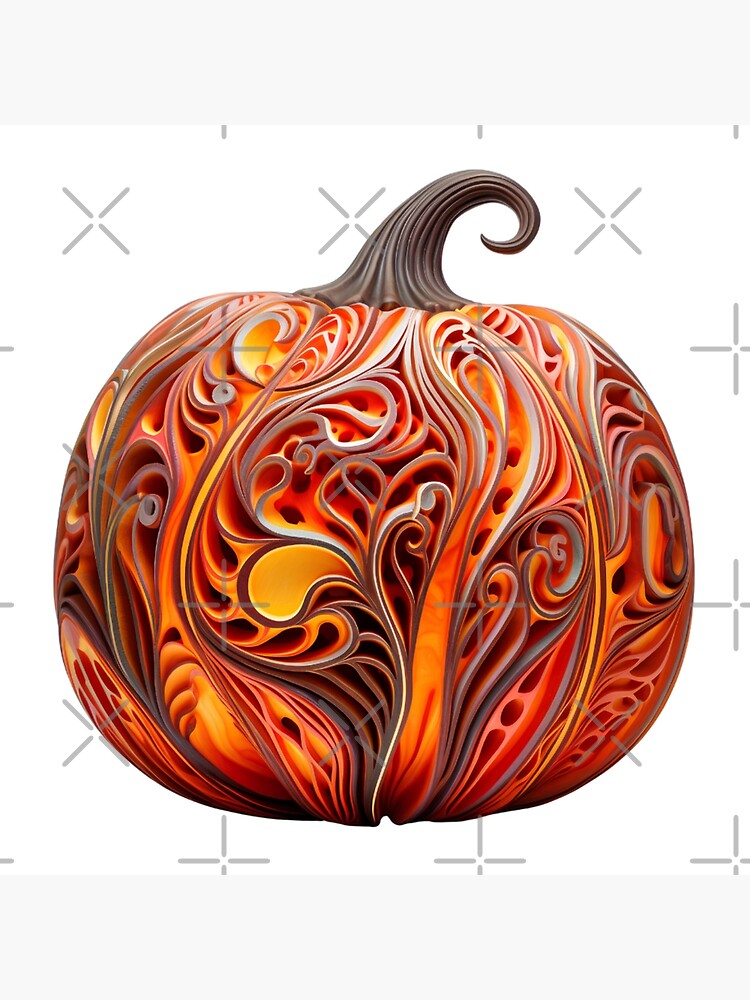This digital illustration features a meticulously carved pumpkin centered in the image. The pumpkin, appearing almost computer-generated, showcases ornamental carvings that run deeply across its surface, forming intricate, leaf-like and floral patterns with long, tendril-like structures. These carvings, primarily light gray, contrast beautifully with the pumpkin's glowing hues of light orange, dark orange, yellow, and gray, creating a sense that it is lit from within. The stem, a brownish-gray hook-like structure, tilts to the right and curls inward at the top. The background is white, adorned with X and plus shapes in gray, blending seamlessly with the pumpkin’s elaborate designs. This sophisticated and carefully rendered piece exemplifies the ornamental vegetable art style.